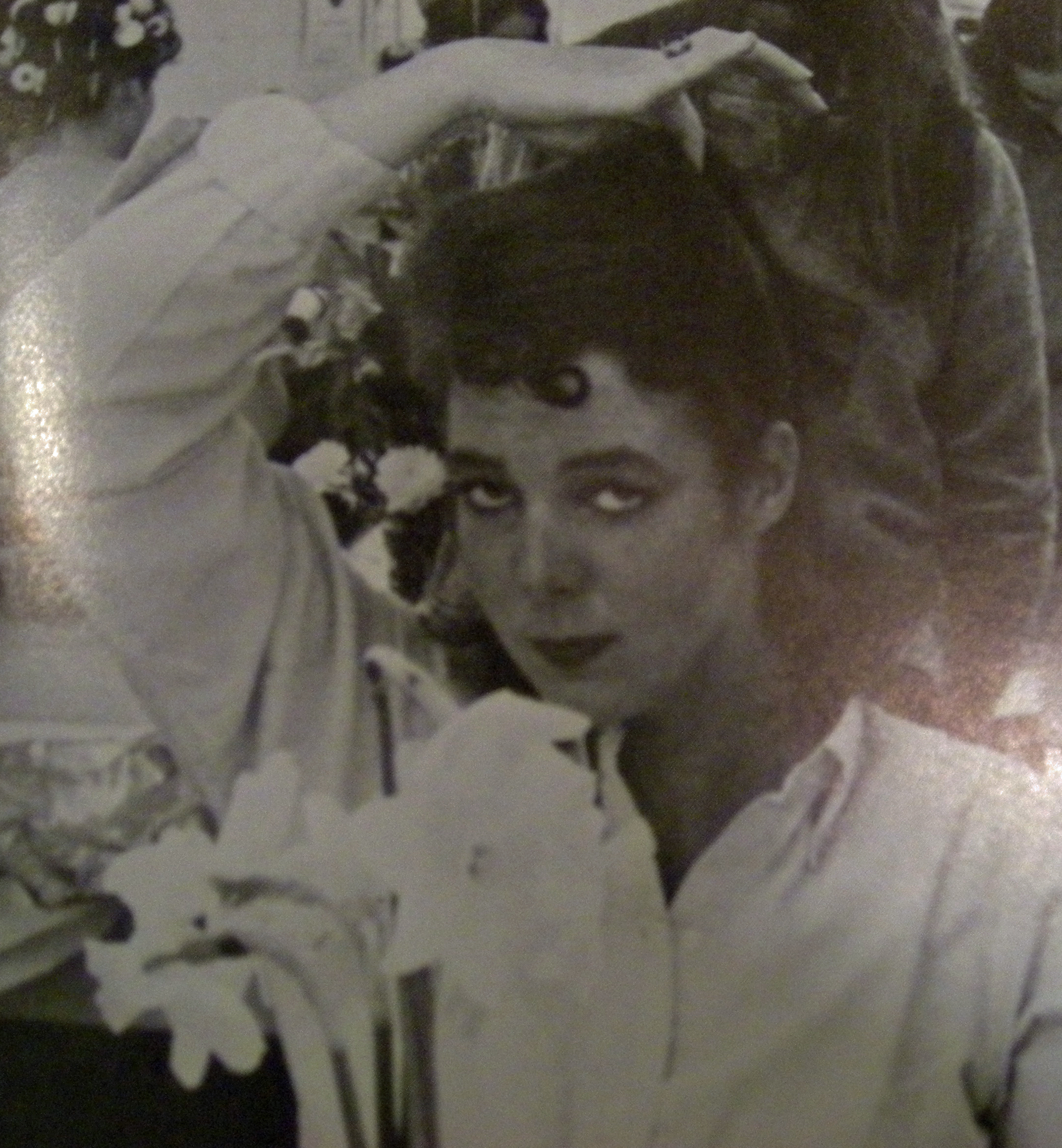This black and white, slightly grainy photograph appears to be an older image of actress Allison Janney, possibly sourced from a yearbook or a vintage periodical. The photograph seems to have been captured by snapping a photo of the original page, resulting in some glare on both the left and right sides of the image. Allison Janney is centrally positioned, with her face directly in the middle and her body leaning slightly towards the bottom right corner. She is wearing a white blouse and dark lipstick, though the exact color can't be determined due to the black and white nature of the photo. Her dark hair features a small curl on her forehead and is pulled up into a ponytail by her right hand, forming a triangle with her arm. In the background, other individuals are faintly visible, some possibly wearing sweaters and curlers in their hair, suggesting a casual or preparatory setting. White flowers are positioned in front of Allison, adding a touch of contrast to the monochromatic scene.